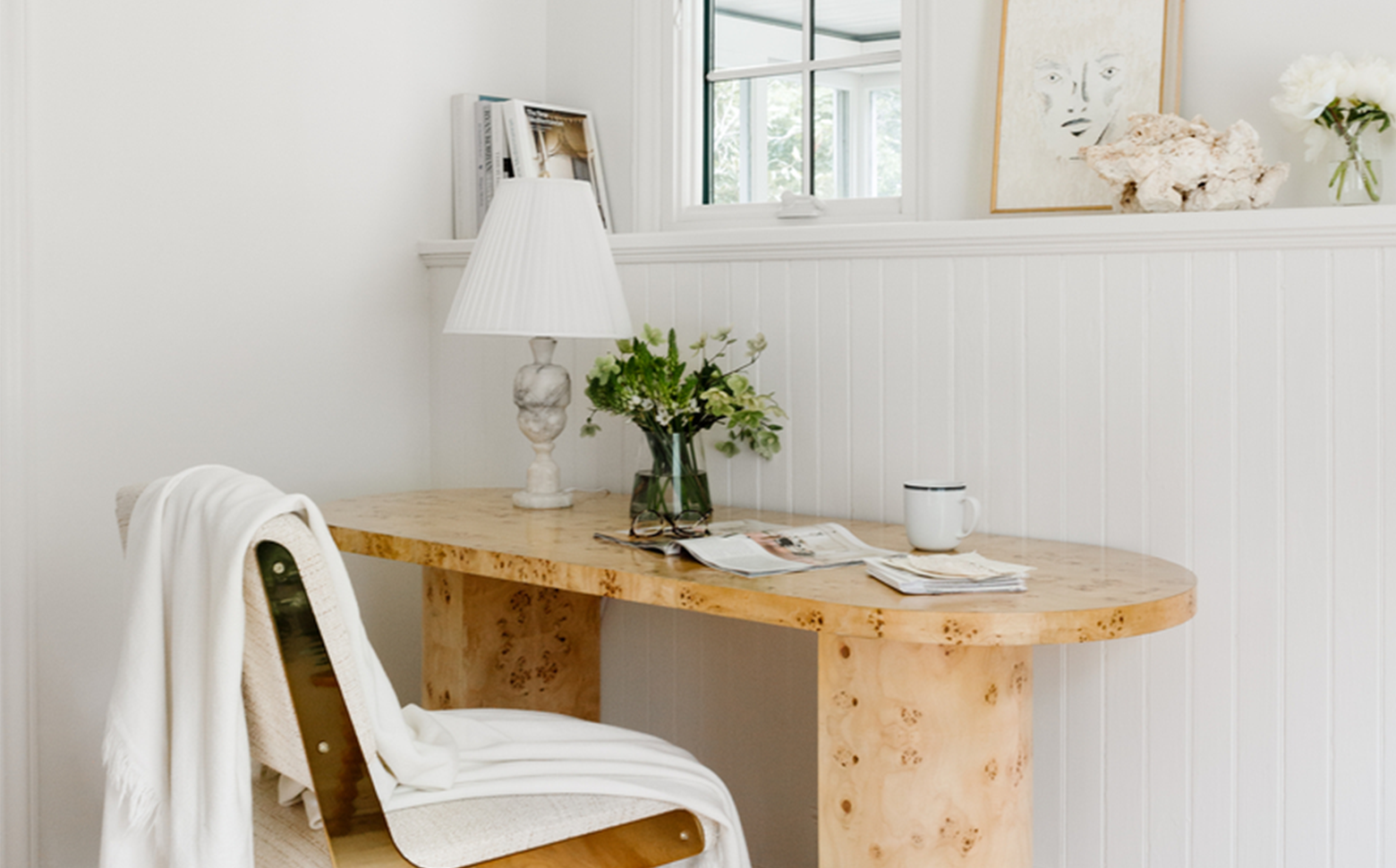This image is a horizontally aligned color photograph of a cozy, feminine work nook in a house, featuring a modern yet inviting aesthetic. The focal point is an oval-shaped desk with a light beige surface accented by a dark brown speckled tortoise shell effect, supported by two solid vertical wooden supports. The desk is centered against a short section of white paneled wall, with a small window nestled above it that brings natural light into the space.

On the desk, from left to right, there's a silver lamp with a white shade, providing gentle illumination to the area. In the center, a clear glass vase holds some fresh white flowers accented with green leaves, adding a touch of natural beauty. Adjacent to the vase, a white coffee mug with a silver rim rests on the right side of the desk, alongside a few scattered documents, suggesting a space used for both work and relaxation. 

To the left of the desk, a chair is partially pulled out, featuring dark wood accents and draped with a white blanket, complete with fringe that cascades softly over the edges, enhancing the snug atmosphere. Above the desk, a built-in shelf holds a tasteful arrangement of items, including a picture frame, a large conch shell, and more white flowers, further adding to the room's serene and elegant style. The predominant color scheme is white, giving the space a clean and cohesive look, with an overall style that blends photographic realism with practical warmth.